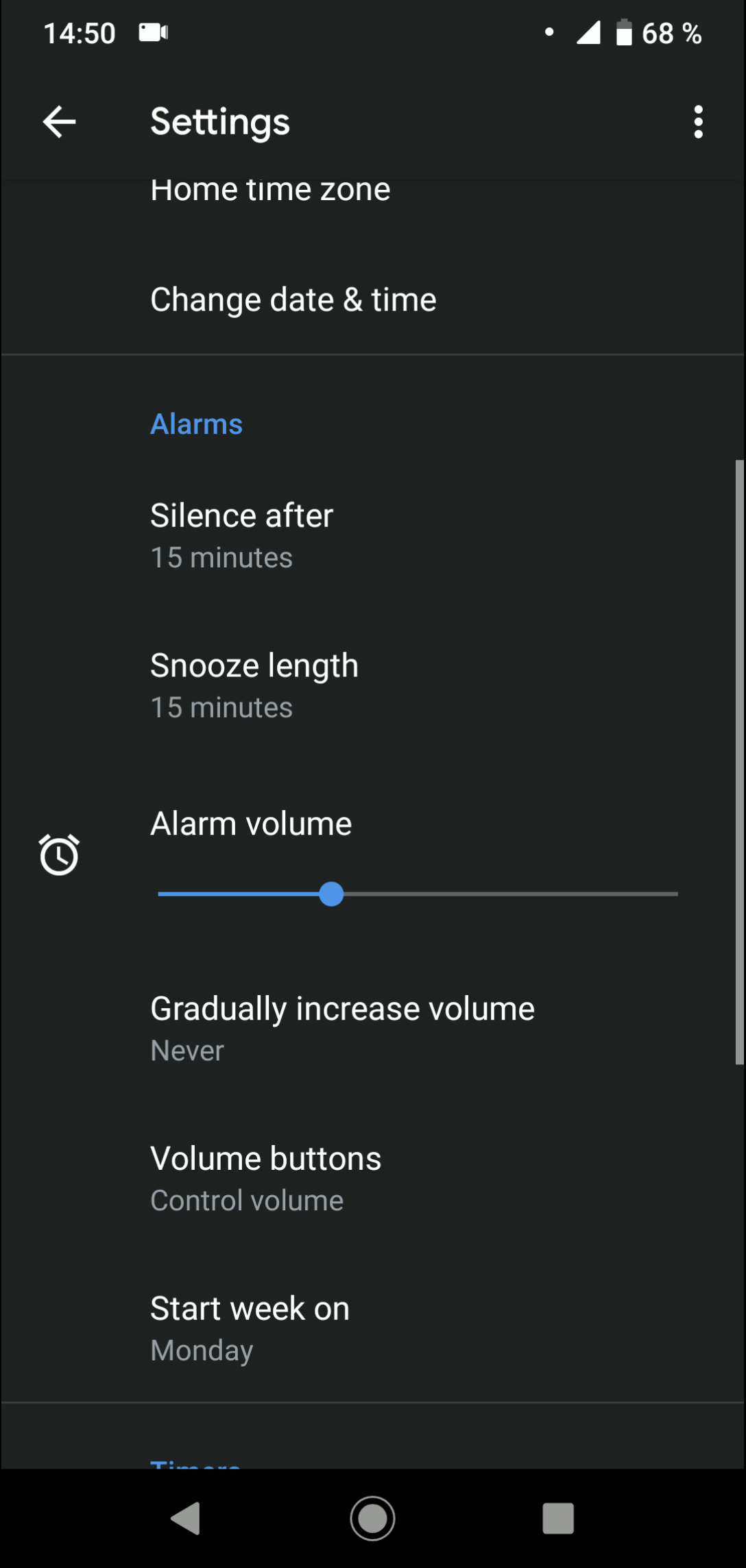This image is a screenshot of a cell phone settings application, featuring a structured layout with various options. 

### Header:
- Dark grey header with:
  - Time displayed as "1450" in white text,
  - A white movie camera icon to the right of the time,
  - A series of icons on the right: a white dot, a white triangle, a battery icon showing 68% with a white bar, and the battery percentage "68%".

### Navigation Bar:
- Beneath the header, a navigation bar contains:
  - A white left-pointing arrow on the left,
  - The bold word "Settings" centered,
  - Three vertically stacked white dots on the far right.

### Body Content:
- The body of the page has a slightly lighter grey background, separated from the header by a dark grey line.
- The settings options are laid out in rows of white text, each option slightly indented:
  1. **Home time zone**
  2. **Change date and time**

- Below these, a light grey line separates:
  3. **Alarms** (displayed in blue text)

- Following options with white text and grey subtext:
  4. **Silence after**: "15 minutes"
  5. **Snooze length**: "15 minutes"
  
- **Alarm volume** setting displaying:
  - A bar indicating volume level, approximately one-third filled with a blue line,
  - A blue circle indicating the point where the blue and grey meet,
  - To the left, a white clock icon centered between "Alarm volume" and the volume bar.

- Following options:
  6. **Gradually increase volume**: "Never"
  7. **Volume buttons**: "Control volume"
  8. **Start week on**: "Monday"

Each segment of the settings UI is clearly demarcated with negative space and light grey separating lines, ensuring a clean and user-friendly interface.